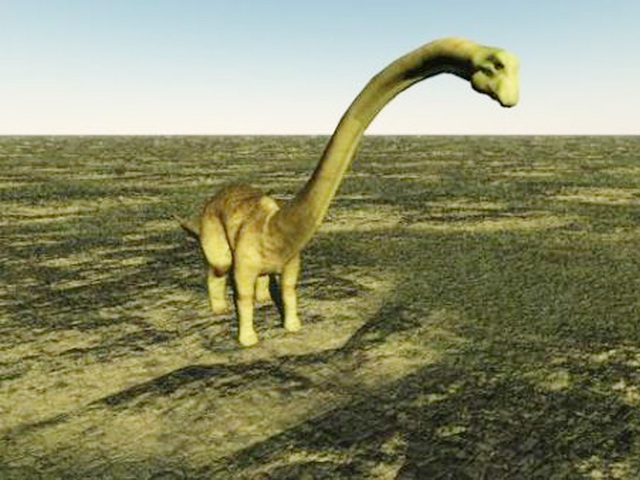This is a detailed artist's rendering of a large, green dinosaur standing on a vast plain, taking up about two-thirds of the image. The dinosaur, presumably a sauropod with traits similar to a plesiosaur or other long-necked dinosaur, is centrally positioned and depicted in various shades of green. It possesses an extraordinarily long neck with a pointed, snake-like head, short front legs compared to its massive back legs, and a very long tail. The surrounding terrain appears from above to be either grassy land or the tops of trees, depicted in greens and yellows. The sky above transitions from a light blue at the horizon to a darker blue at the top, contrasting with the dinosaur's imposing height. Despite the dinosaur’s enormous and somewhat imposing figure, it appears benign, calmly surveying the expanse of minimal vegetation that stretches endlessly to the horizon. The image emphasizes the dinosaur's unusual and impressive natural features, highlighting the fascination and creativity of the artist's interpretation.